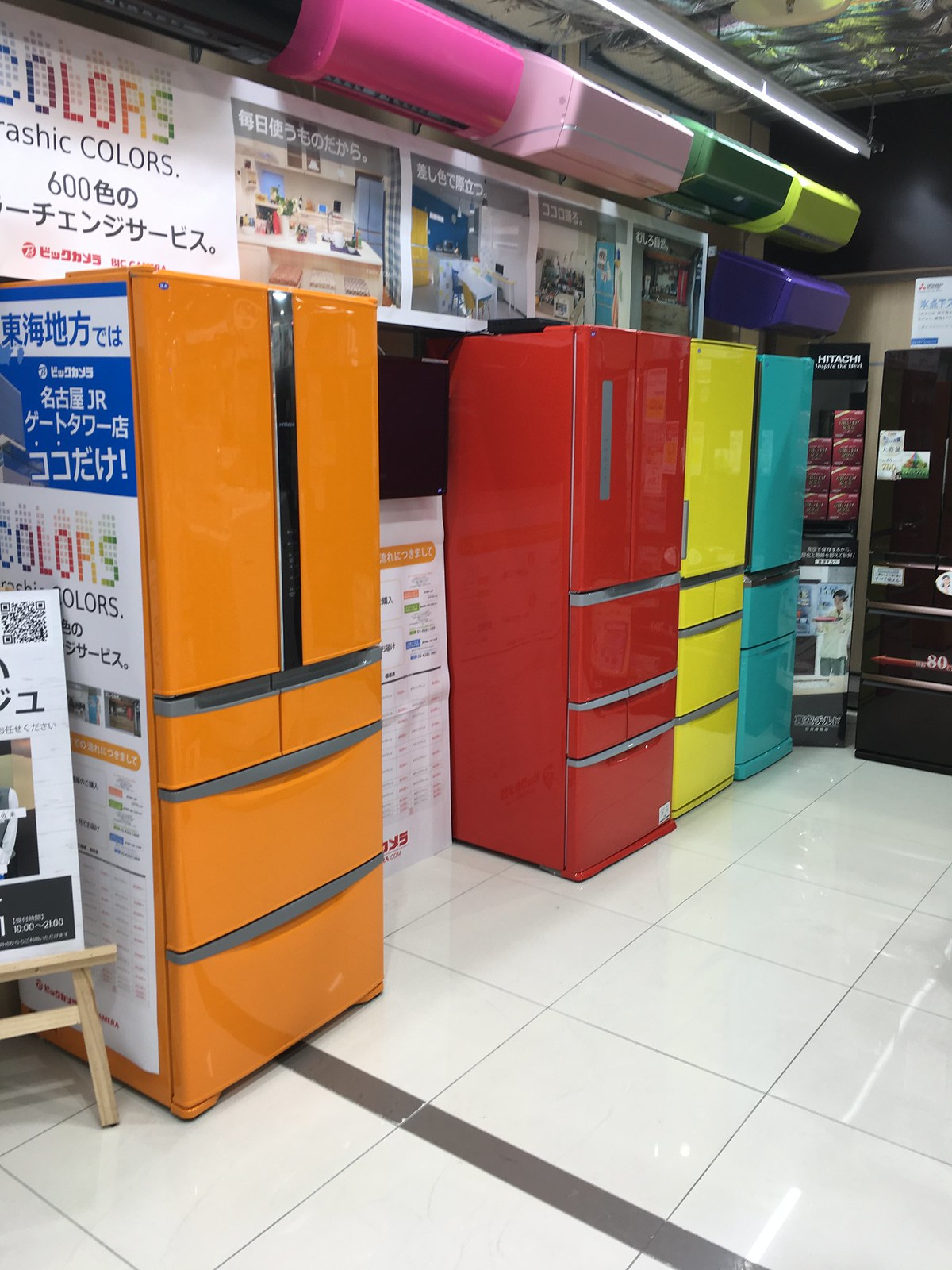This photograph captures the inside of a furniture supply store, with most of the text on the store's banner displayed in an Asian font, possibly Chinese, and a prominent heading in bright, bold colors. The banner partially reads "600" amidst other unreadable text and displays images of various furniture arrangements. Positioned on a polished white ceramic tile floor that reflects the overhead fluorescent lights, there is a row of five distinct refrigerators against the wall. These appliances come in vibrant colors: orange, red, yellow, turquoise, and black. Each refrigerator features gray handles etched into the doors, with some having split drawers beneath them. In front of the foremost refrigerator stands an easel holding an advertisement poster, also written in Asian text. Above the refrigerators are colorful vent AC units in teal, lime, hot pink, pink, purple, and black, adding to the store's eclectic mix of colors.